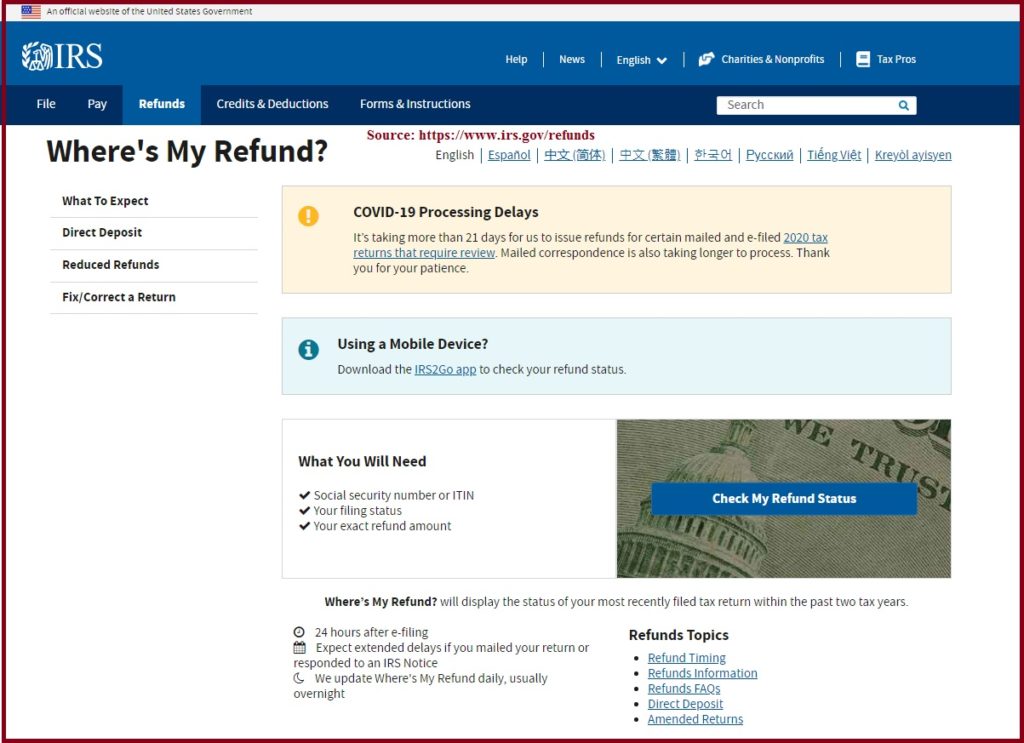This is a detailed description of a screenshot from the IRS website. The image is bordered by a bold red rectangle. At the very top, there is an image of an American flag accompanied by the text, "An official website of the United States government." Just below this is a dark blue header displaying the IRS logo and name. This header includes several navigation tabs: File, Pay, Refunds, Credits & Deductions, Forms & Instructions, as well as further options for Health, News, Charities & Nonprofits, and Tax Pros, located on the right side of the header. There is a search bar in the lower right corner of the rectangle.

On the left side of the screen, there’s a vertical column listing several links: "Where's My Refund," "What to Expect," "Direct Deposit," "Reduced Refunds," and "Fix, Correct, or Return."

The right two-thirds of the screen are segmented into multiple rectangles. The first section is about COVID-19 processing delays, highlighted in a yellow rectangle, informing users that it is taking more than 21 days to issue refunds for certain mailed and e-filed 2020 tax returns requiring review. It also notes delays in processing mail correspondence and thanks users for their patience.

Below this is a light blue rectangle with guidance for mobile device users, suggesting they download the IRS2Go app to check their refund status. Further down, in a white rectangle, there is a list titled "What You Will Need," detailing the requirements to check your refund status: Social Security number, filing status, and exact refund amount. Adjacent to this list is an image of part of a dollar bill with a button labeled "Check My Refund Status."

At the bottom of the section, there is information about the "Where's My Refund" service, explaining that it will display the status of the most recently filed tax return within the past two years and that status updates are typically available 24 hours after e-filing. It also mentions that there may be extended delays for mailed returns or responses to IRS notices, with daily updates usually occurring overnight. Additional topics addressed include refund timing, refund information, refund facts, direct deposit, and amended returns.